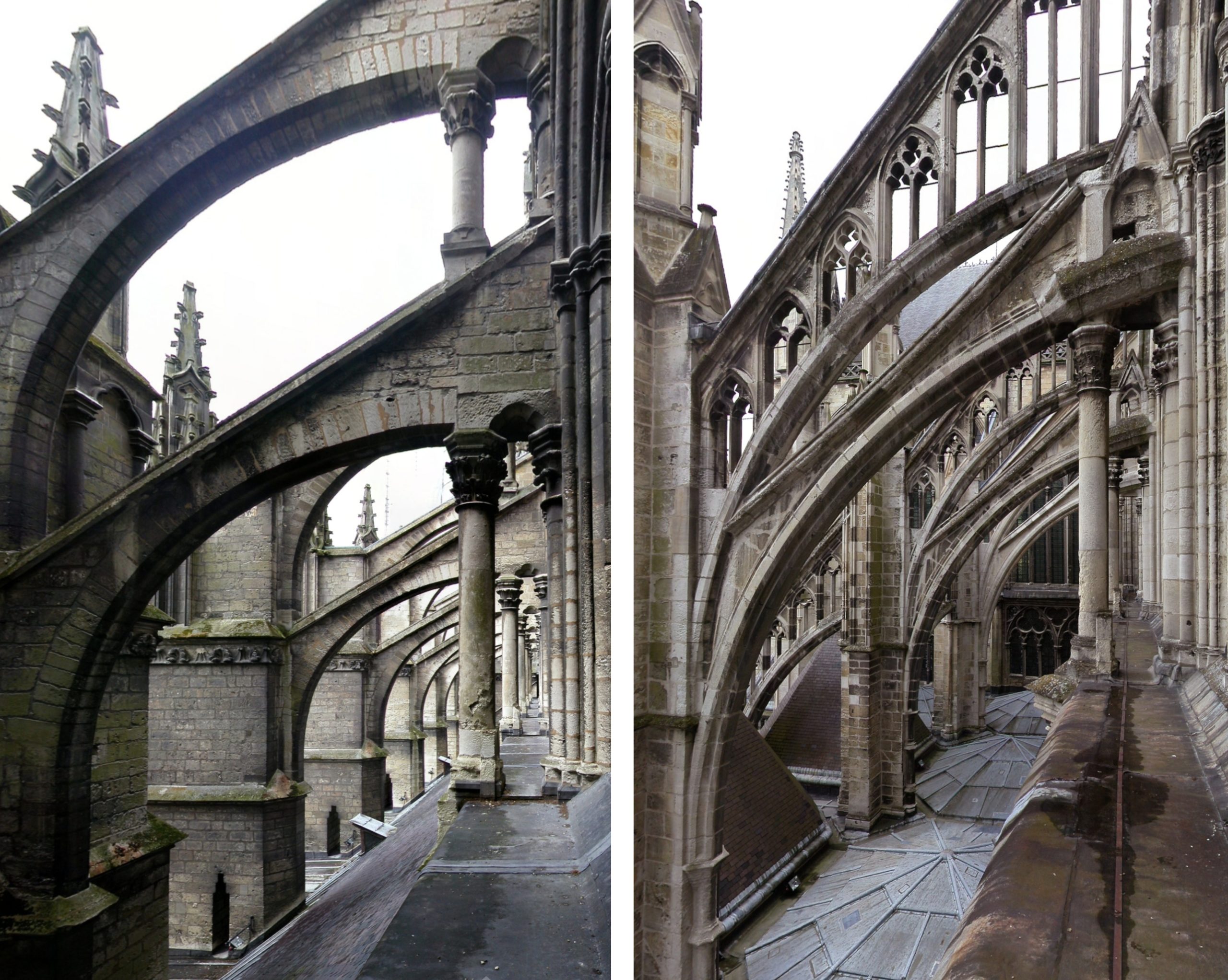The two side-by-side images depict a grand and ancient stone building, reminiscent of European Renaissance church architecture. Both images showcase towering stone arches, intricate columns, and detailed designs that hint at windows and decorative elements. The right-hand image captures two prominent arches supported by pillars, with three steeples visible in the background. The left-hand image reveals a series of arches leading to a pathway adorned with domed windows and circular motifs. Both scenes are set against a bright, washed-out, overcast sky, lending a timeless and serene ambiance to the composition. There are no people present in either image, allowing the viewer to fully appreciate the architectural beauty and historical essence of the structure.